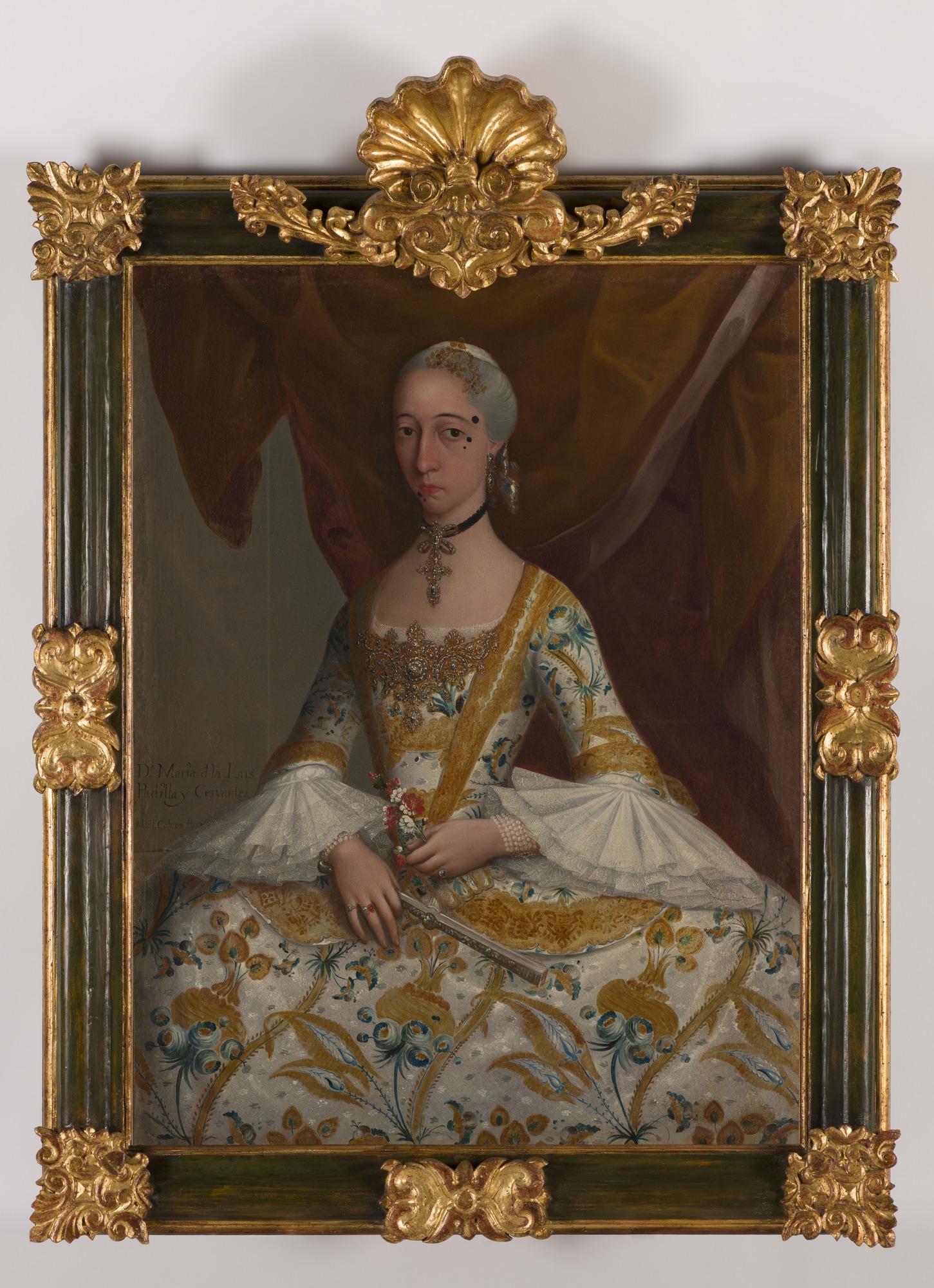This image depicts a professionally taken photograph of a painting of a white woman with short gray hair, seated for a portrait. She is dressed in an elaborate Victorian-style gown that features an intricate pattern of gold lamé and floral designs, including gold flowers with blue stems and leaves. The bodice of her dress is ornate, embroidered, and beaded, with gold lines running from her shoulders to her belly button. The sleeves are tight to the elbows and flare out into white lace frills. She wears a choker necklace with an emblem and ornate dangling earrings, and her hair is pulled back tight with a small cap. Her face bears thin, arched eyebrows and notable black moles. She holds a small bouquet of red and white flowers in her left hand. Behind her is a mustard-colored curtain. The painting is encased in a very detailed greenish-gold wooden frame, featuring floral embellishments at each corner, the middle of the sides, and a large ornate emblem at the top. The gold gilding and dark enamel give the frame an antique, sophisticated appearance.